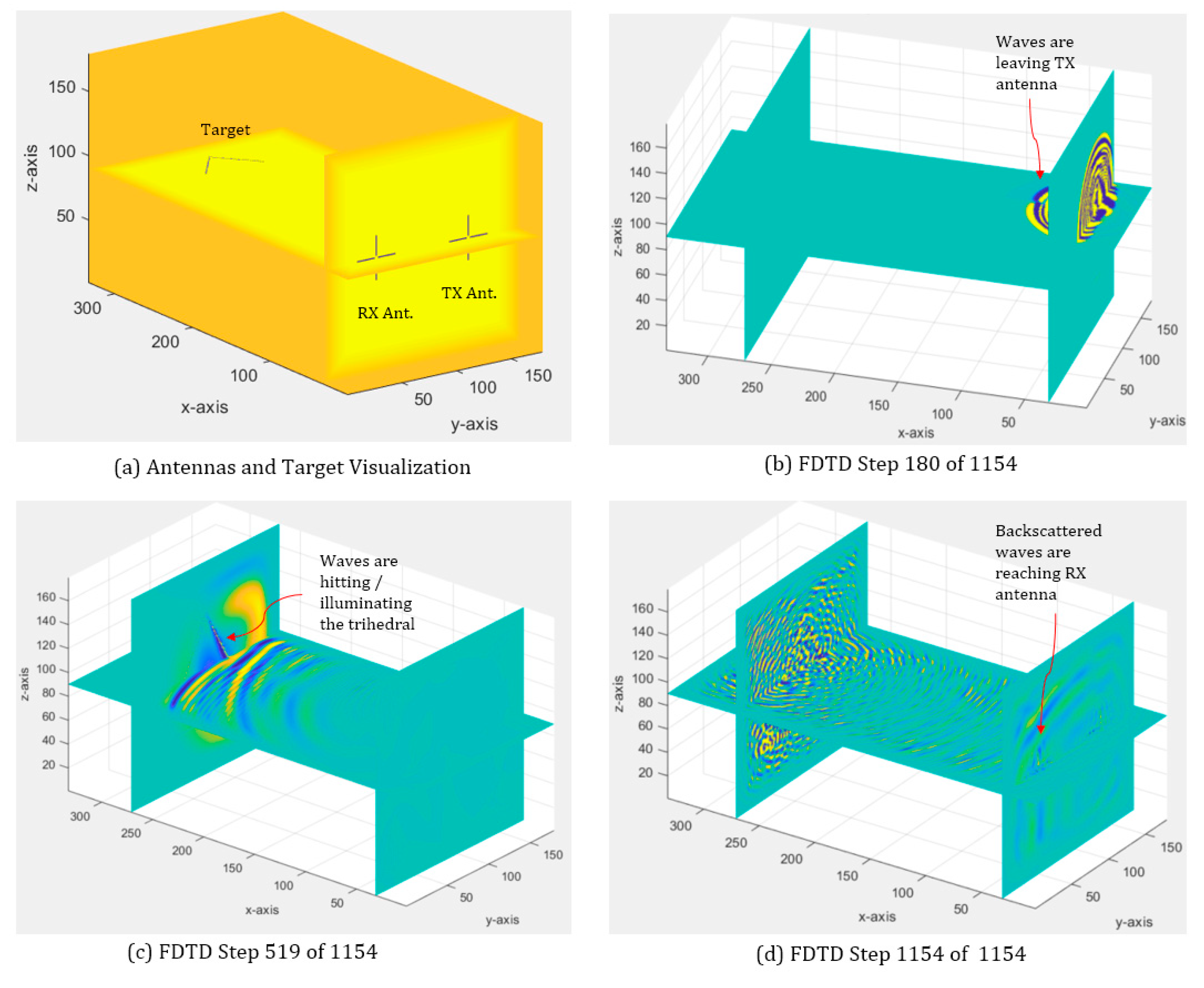This image is a collage of four detailed diagrams labeled A, B, C, and D, each illustrating different steps in an antenna simulation process. 

In the top left corner, Diagram A, titled "Antennas and Target Visualization," features a nearly rectangular orange object with a yellow interior, surrounded by numbers on the left, bottom, and right sides. The axes are labeled z-axis on the left, x-axis and y-axis at the bottom. This diagram likely shows the initial stage of the simulation.

To the right, Diagram B shows a clear white rectangular box intersected by horizontal turquoise lines, labeled as "FDTD Step 180 of 1154." This step demonstrates the intermediate phase in the simulation process.

In the bottom left, Diagram C, also a clear white rectangular box, is labeled "FDTD Step 519 of 1154." It illustrates a further advanced stage in the simulation.

Finally, the bottom right, Diagram D, labeled "FDTD Step 1154 of 1154," shows the final stage of the simulation. 

These series of images depict the progression of the finite-difference time-domain (FDTD) method being applied to model the behavior of electromagnetic waves emitted from an antenna as they interact with and illuminate a target object, eventually backscattering and re-reaching the antenna.